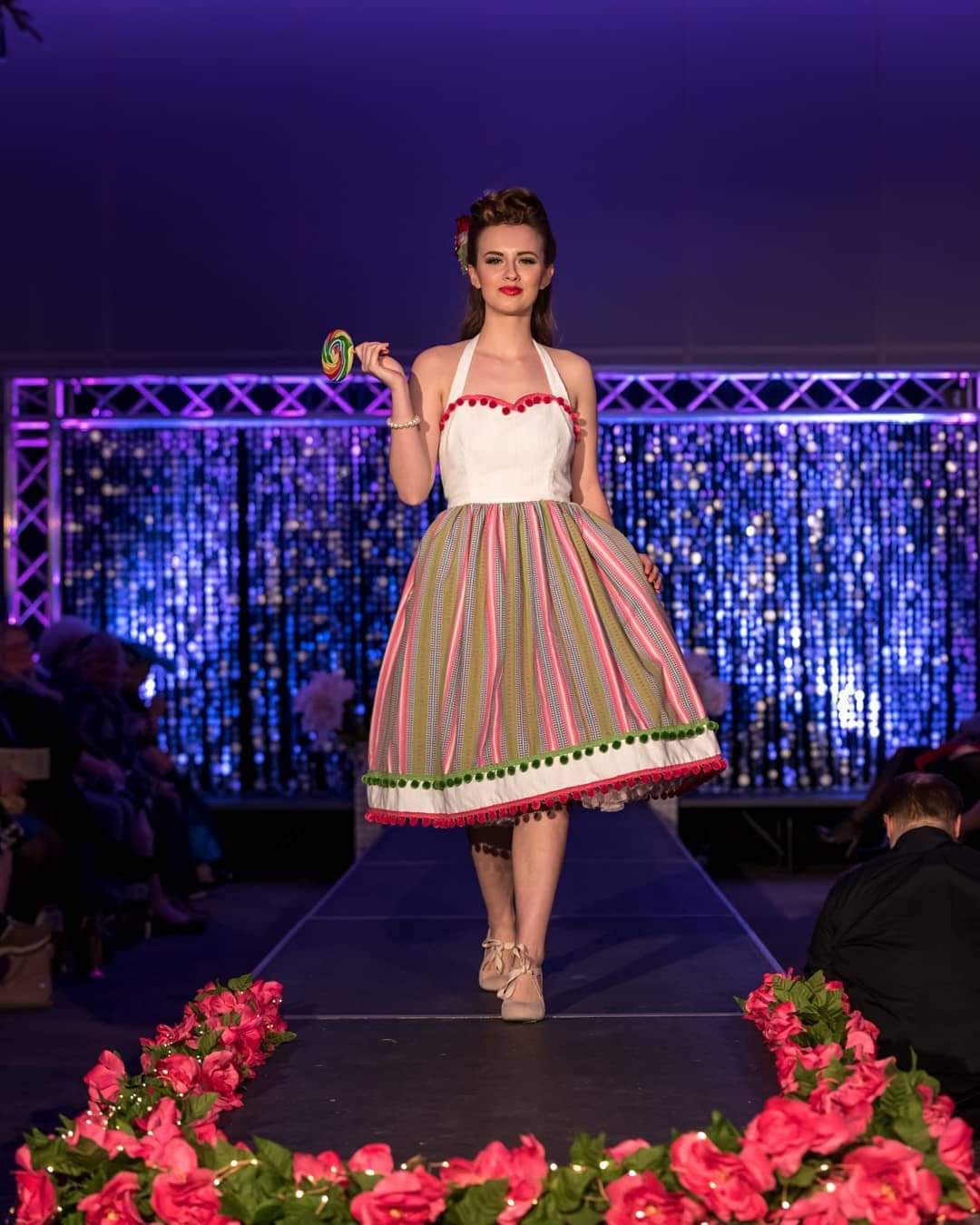In the photograph, a woman walks confidently down a short fashion walkway, which extends from a stage adorned with a blue wall and a shimmery blue and purple glittery curtain. The stage backdrop includes a metal structure with bluish and yellowish decorative elements. The walkway itself is dark, bordered by pinkish-red roses arranged in a U-shape, and the surroundings are dimly lit, making it difficult to distinguish the seated audience.

The woman, who has light brown hair partly pulled back with flowers adorning the right side, is dressed in a 1960s-inspired summer dress. The dress features a white bodice with red pom-pom trim and white straps, transitioning into a poofy, striped skirt in shades of green, red, white, and black. The skirt is accented by a green trim with green pom-poms, a white strip, and finally, a red trim with red pom-poms. Complementing her outfit, she wears beige ballet slippers. In her right hand, she carries a multicolored swirly lollipop, while her left hand delicately holds up her skirt, her demeanor cheerful and slightly smiling.